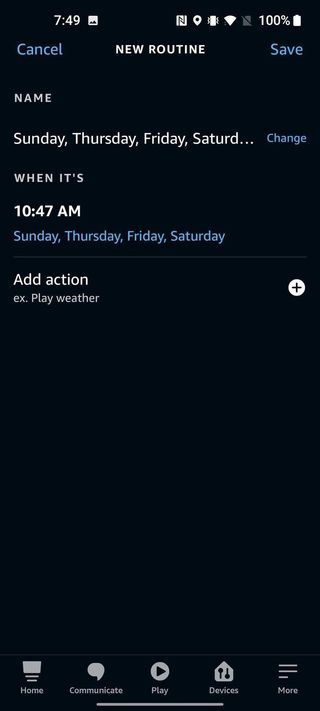This image depicts the screen of a device, likely a smartphone or tablet, with various interface elements displayed. In the top-left corner, the time is shown as "7:49" next to a picture icon. The top-right corner features several status icons, including those for GPS, vibrate, Wi-Fi, and a battery icon indicating 100% charge.

Below the status bar, the screen is divided into three main sections. The top section, from left to right, displays the options "Cancel," "New Routine" in the center, and "Save" on the right. Immediately below this section, there is a field labeled "Name," followed by a row of days: "Sunday, Thursday, Friday, Saturday," with a "Change" option adjacent to it.

The next section displays the label "When It" with the time "10:47 AM" beneath it. This is followed by another row listing the days "Sunday, Thursday, Friday, Saturday."

Further down, there is an "Add Action" option with an example action "EX.PlayWeather." To the far right of this option is a plus button, presumably for adding new actions.

At the very bottom of the screen, there are several tabs, with the first labeled "Home," indicating the presence of a navigation bar.

Overall, this screen appears to be part of a scheduling or routine-setting application, with detailed fields for specifying days and times as well as customizable actions.